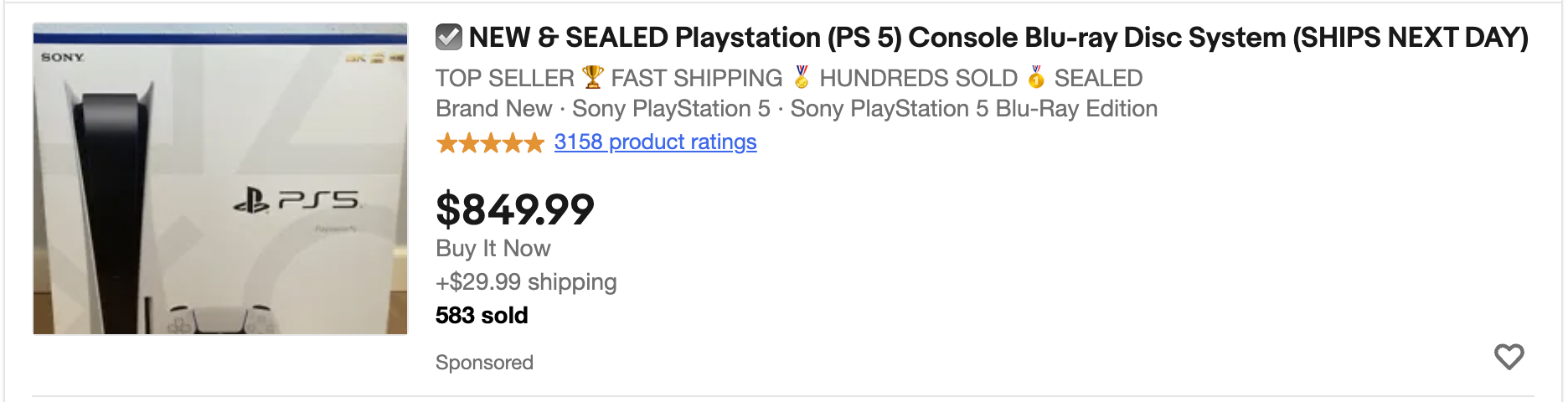This image is a screenshot of an online product listing for a Sony PlayStation 5 console, presented within a border outlined by a light gray line that runs from the bottom left to upper left, upper right, and then to the lower right. The border has small gaps at the bottom left and bottom right corners. 

On the left side of the screenshot, there is a white Sony PS5 box prominently displayed. Overlapping the box image is a black stick featuring the title "New and Sealed PlayStation PS5 Console," indicating the product condition. Below this title, the listing showcases various award icons including a "Top Seller Award," "Fast Shipping Award," and "Hundred Sold Award Seal."

Further down, the product description reads "Brand-New Sony PlayStation 5," specifying that it includes the "Sony PlayStation 5 Blu-ray Edition." The product has received an impressive rating of 5 out of 5 stars based on 3,158 reviews, with the rating section appearing as a clickable blue link. 

The price of the console is listed at $849.99 with an additional $29.99 for shipping, and it is noted that 583 units have been sold. In the bottom right-hand corner of the screenshot, there is a translucent heart icon that can be clicked on to add the item to a favorites list.